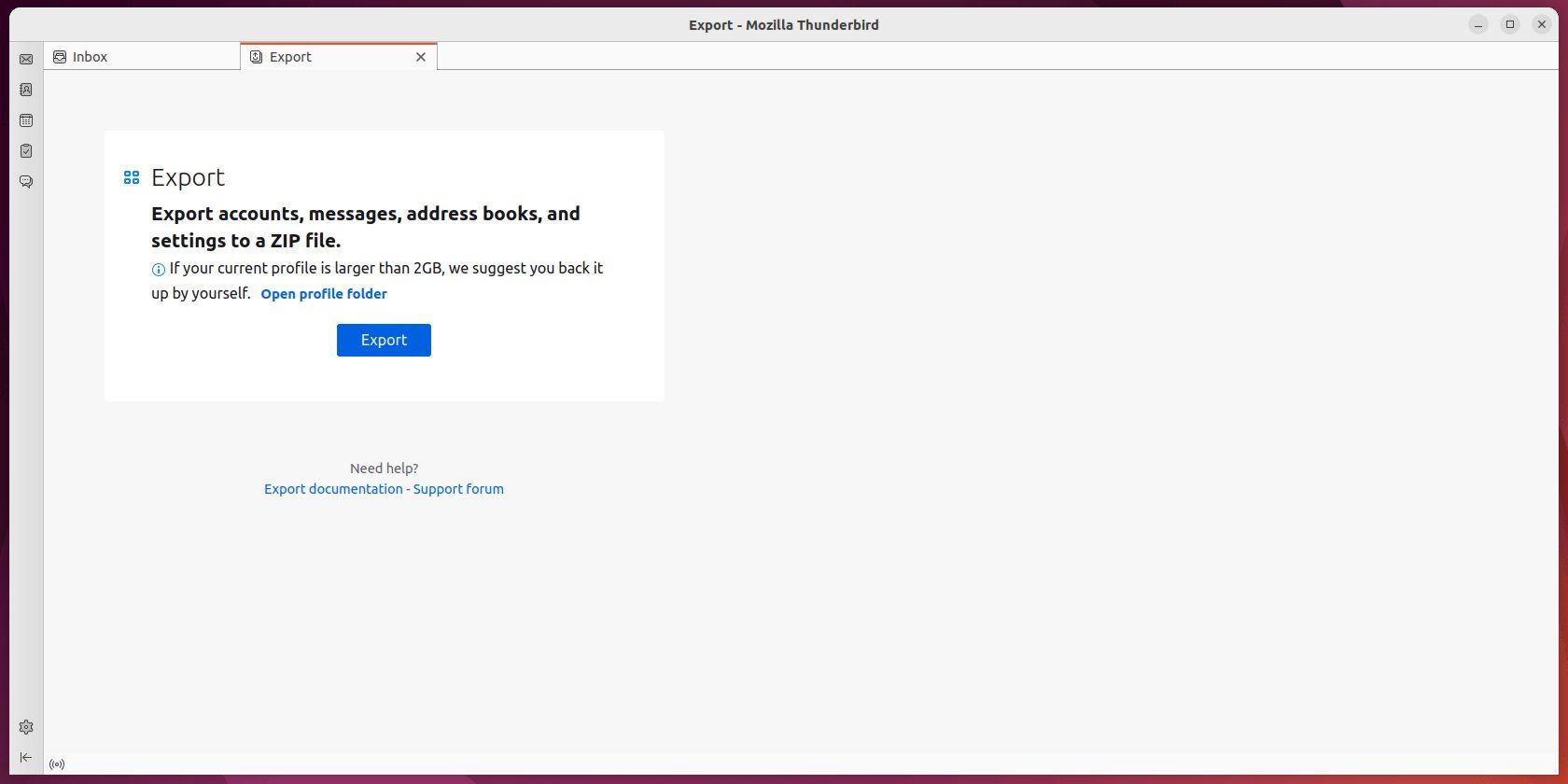The image depicts a user interface screen with a white background and black text, framed by a thin red border. At the top, it features options for exporting data from Mozilla Thunderbird, such as inbox, accounts, messages, address books, and settings, consolidated into a single ZIP file. A note advises users with profiles larger than 2GB to manually back up their data. Below this, there is an "Open Profile Folder" option followed by buttons labeled "Export," "Find Help," "Forgot," "Export Documentation," and "Support." The "Export" button stands out in blue with white lettering, and the "Export Documentation" and "Support" sections share this blue theme. At the top right corner of the screen, there are three familiar window control buttons: Minimize, Maximize, and Close (marked with an "X"). There is also a mention of a "Twoop Forum" and an "Inbox" in the surrounding text.